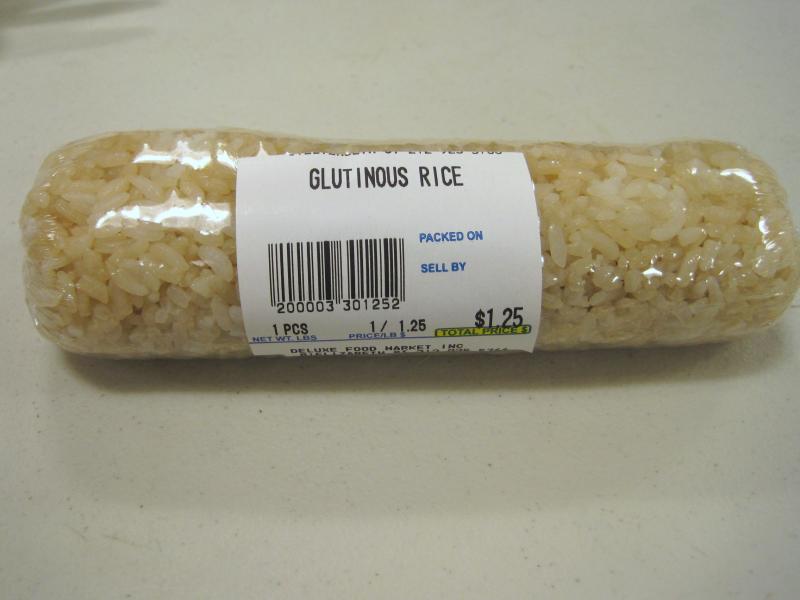This image depicts a close-up view of a packaged product resting on a countertop indoors. The item in focus is a small, cylindrical bag of rice, resembling the shape of a sausage. The label on the package identifies it as "Glutinous Rice." Notably, the label indicates a spot for a packaging date, although no specific date is provided. Similarly, there is no "sell by" date listed. The net weight is specified as one piece (1 PCS), and the price is clearly marked at $1.25.